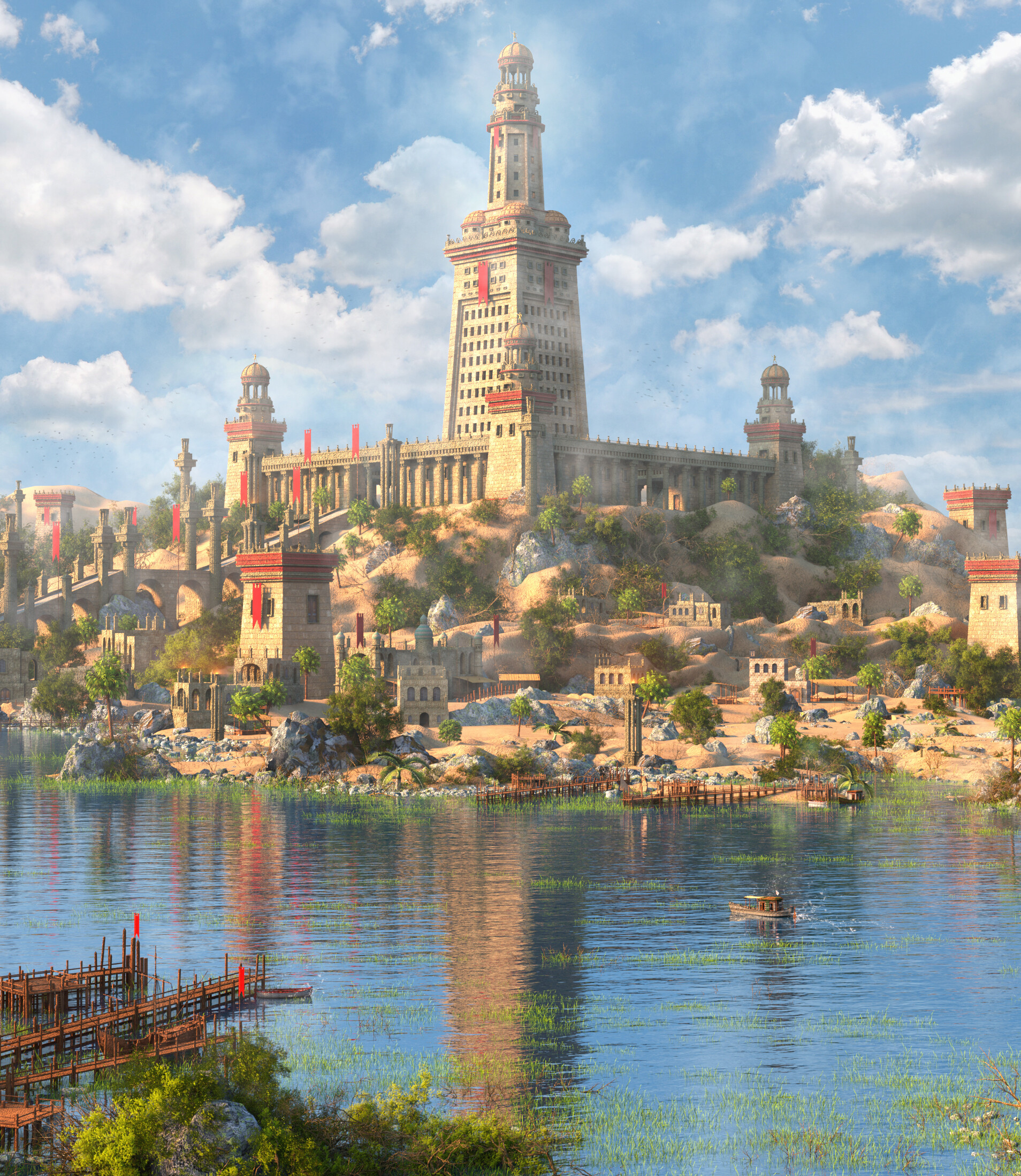The image depicts a 3D illustration with a slight painterly feel, showcasing a grand, fortress-like structure set against a blue sky dotted with light clouds. At the center of this fortress, there is a towering square bell tower crowned with a dome. Surrounding the central tower are robust walls, each corner fortified with small domed watchtowers adorned with red flags fluttering above.

The facade of the building, characterized by pillared sides, is reached by a long staircase that ascends in segments, flanked by additional pillars and more flags. This staircase extends from the main entrance and adds a majestic approach to the fortress.

In the foreground lies a tranquil body of water—presumably a river—speckled with green lily pads or reeds, adding a touch of nature to the scene. Along the shoreline, both near and across the water, several wooden docks stretch into the river, hinting at the river’s utility for the town.

Scattered across the rocky hillside leading from the towering fortress down to the water are smaller stone buildings, likely part of a village that appears deserted, with only a few trees and some brush dotting the landscape. The composition combines elements of natural beauty and architectural grandeur, creating a detailed and immersive scene.